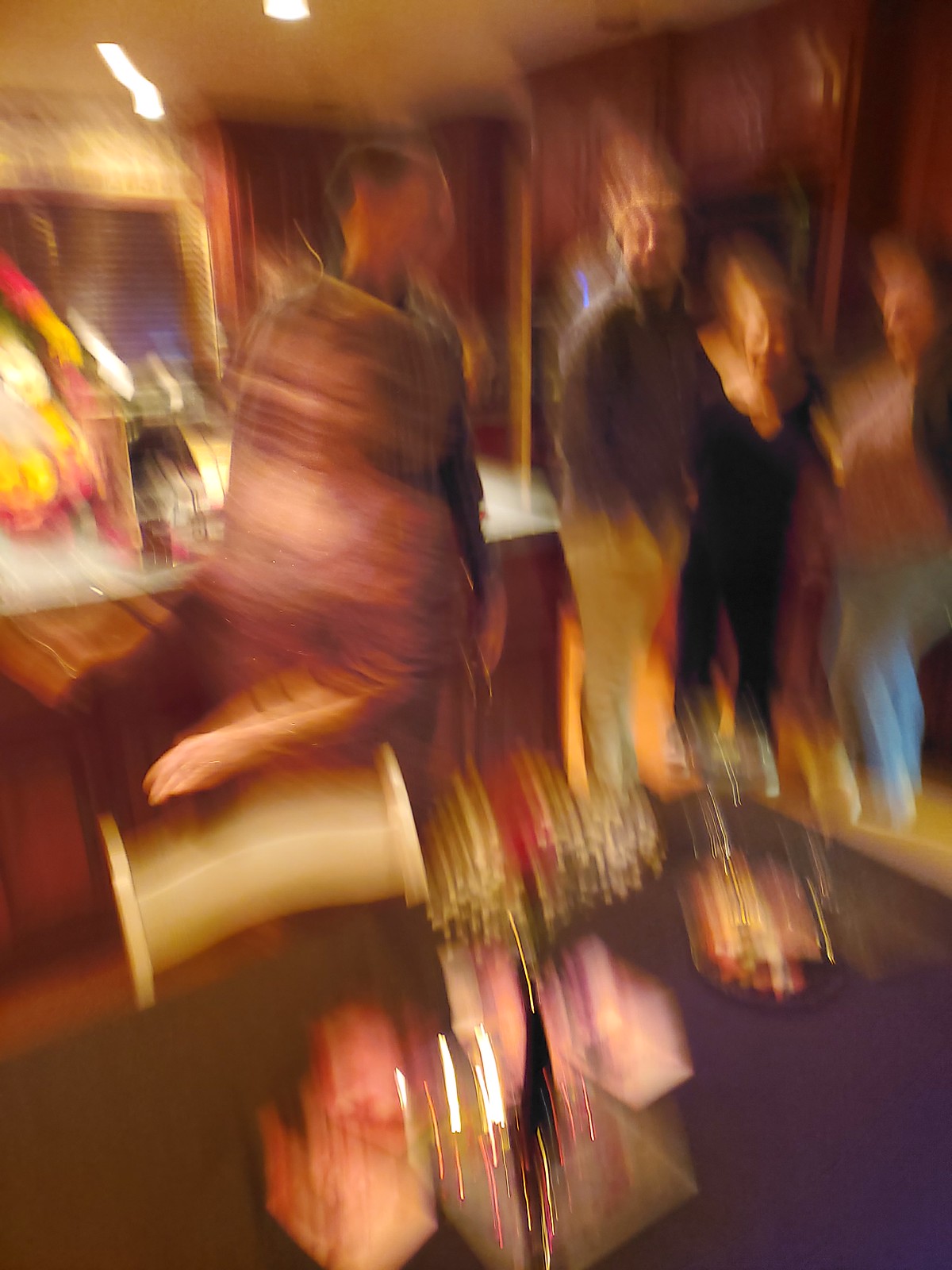The image appears to be a heavily distorted and blurred scene, suggestive of an artistic or perhaps unintentional photographic effect. It captures a lively gathering, potentially in a kitchen or dining room setting. The background reveals four to five people, some more distinguishable than others. Most notably, there is a man with short dark hair in a dark shirt. Nearby, another man with short hair in a dark shirt and light pants stands alongside a shorter woman with short hair, dressed in a black top, black pants, and white shoes. Another person beside her is indiscernible in gender, clad in a combination of dark and white tops and jeans.

The setting includes warm brown wooden cabinetry, possibly incorporating a mounted microwave, and an island with a white granite countertop. The table in the foreground is cluttered with various indistinguishable items, though there appears to be a plate with vegetables like carrots and cheese, as well as flowers, and a white chair. Amidst the blur of colors and shapes, one figure stands out, moving quickly towards the left of the picture with a smile, perhaps preparing food. The overall ambiance is a mix of abstract, almost computer-generated shapes, evoking a funky, arty feel.